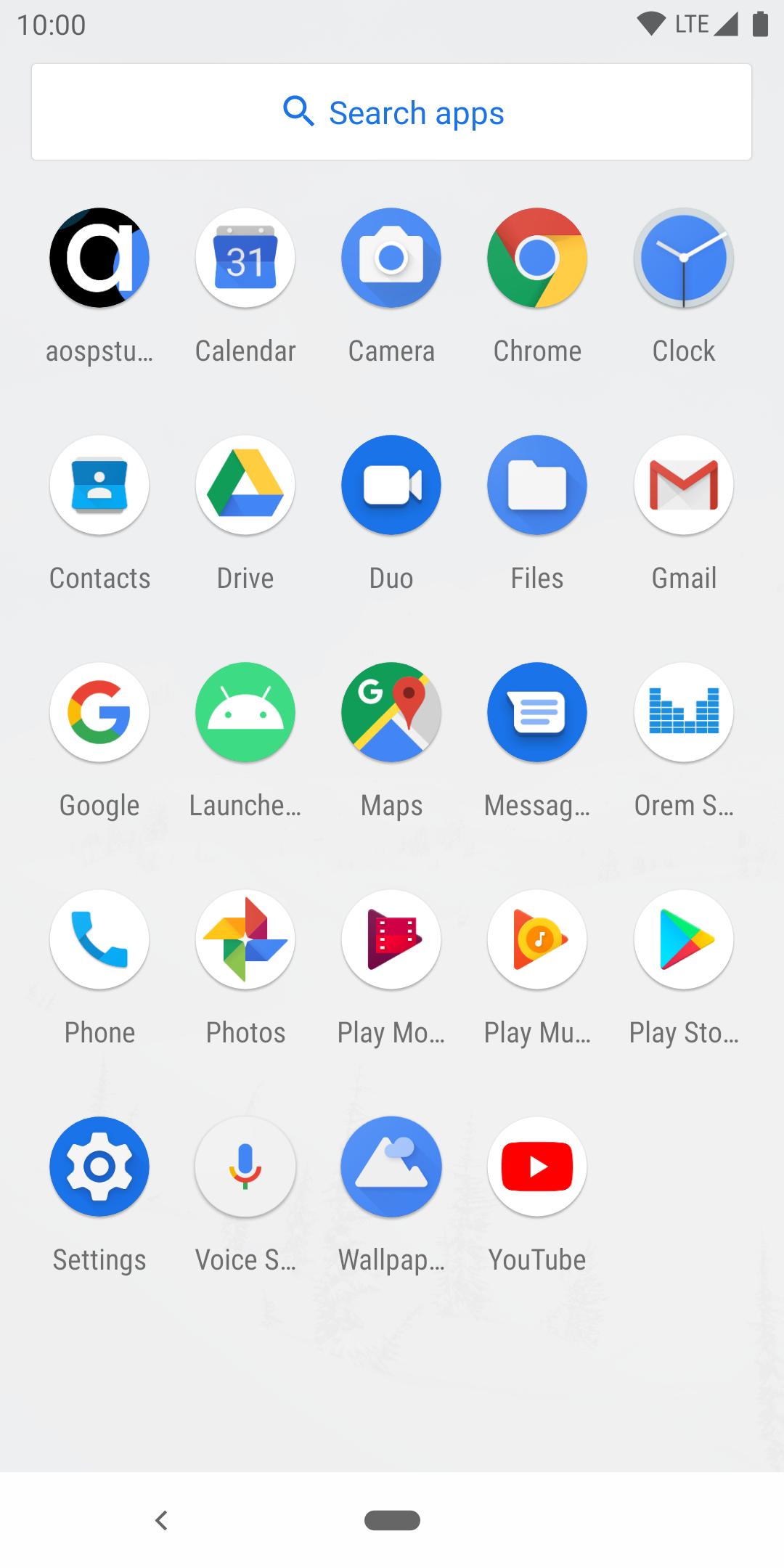This image appears to be a screenshot taken from an Android smartphone. The status bar at the top shows the time as 10:00, a full Wi-Fi signal icon, LTE connectivity, full phone signal bars, and a full battery icon in black. Below the status bar is a search bar with a white background, containing the text "Search apps" and an icon resembling a microscope.

Underneath the search bar, various app icons are displayed in a grid layout. The visible apps include:

1. **AOSPS.TU** - An icon with small dots and a circle, predominantly black with some blue elements and a lowercase "a."
2. **Calendar** - Showcases the number "31" within a blue square.
3. **Camera** - Depicted by a camera icon.
4. **Chrome** - Represented by the Chrome browser icon.
5. **Clock** - Features a traditional clock icon.
6. **Contacts** - Displays a person silhouette within a blue square.
7. **Drive** - Marked by the Google Drive triangle icon.
8. **Duo** - Indicated by the Google Duo icon.
9. **Files** - Represented by a file folder icon.
10. **Gmail** - Shows the distinctive Gmail envelope icon.
11. **Google** - Displayed by the Google "G" icon.
12. **Maps** - (partially visible) representing Google Maps.
13. **Messages** - (partially visible) likely the messaging app.
14. **Phone** - (partially visible) indicating the phone dialer.
15. **Photos** - The Google Photos pinwheel icon.
16. **Play Store** - (partially visible) indicating the Google Play Store.
17. **Settings** - (partially visible) represented by a cogwheel.
18. **Voice** - (partially visible) likely the Google Voice app.
19. **Wallpapers** - (partially visible) for setting wallpapers.
20. **YouTube** - The recognizable YouTube play button icon.

This layout exemplifies a typical Android home screen, featuring a variety of essential Google apps, communication tools, and the device’s built-in functionalities.